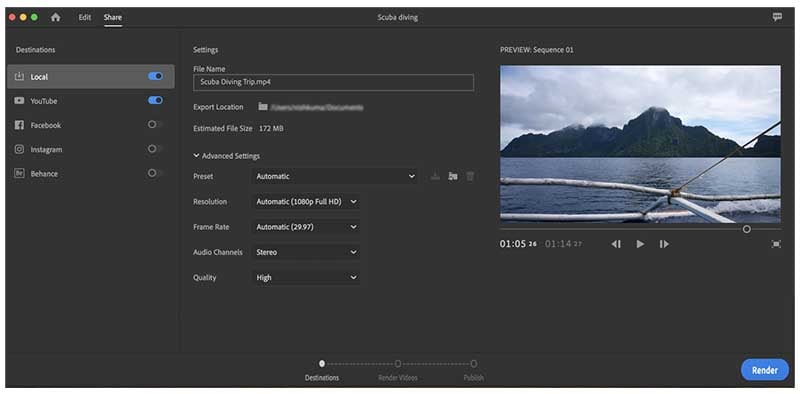This screenshot provides a detailed interface view of a video editing software with a user-friendly design. The screen predominantly features black, with white text throughout.

The center of the screen displays the title "scuba diving" against a black background in a landscape frame format. At the top left, red, yellow, and green dots indicate window controls. Multiple tabs and features are present, including "Icon," "Edit," and "Share," with "Share" being underlined to indicate the active tab.

On the left sidebar, sections labeled "Destinations," "Local," and "YouTube" are displayed. The "Local" and "YouTube" options are highlighted in blue, indicating selection. Other social media options—"Facebook," "Instagram," and "Behance"—remain unselected.

Below this, the "Settings" section includes various details:
- File Name: scuba diving trip.mp4
- Export Location: (blurred out) 
- Estimated File Size: 172 MB
- Advanced Settings dropdown:
  - Preset: Automatic
  - Resolution: Automatic, 1080p Full HD
  - Frame Rate: Automatic, 29.97 fps
  - Audio Channels: Stereo
  - Quality: High

The right portion of the screen features a video preview, titled "Sequence 01." The preview displays a silver metal railing, curving downward toward the right, affixed to a white structure submerging into water. A rope is attached to a rectangular metal bar, possibly associated with the railing. The scene setting depicts a serene body of water, possibly a lake or bay, with a mountain range illuminated in the background. The mountain has a high, centered peak with some white clouds and patches of blue sky.

Additionally, there are timestamps "01:05:24" in white and "01:14:27" in gray, accompanied by standard video controls (rewind, play, forward, and stop). The video's progress bar shows that it is 90% complete.

At the bottom of the screen, options including "Destinations," "Render Videos," and "Publish" are present, with the "Destination" tab highlighted. A blue "Render" button is located at the bottom right, inviting users to finalize their video.